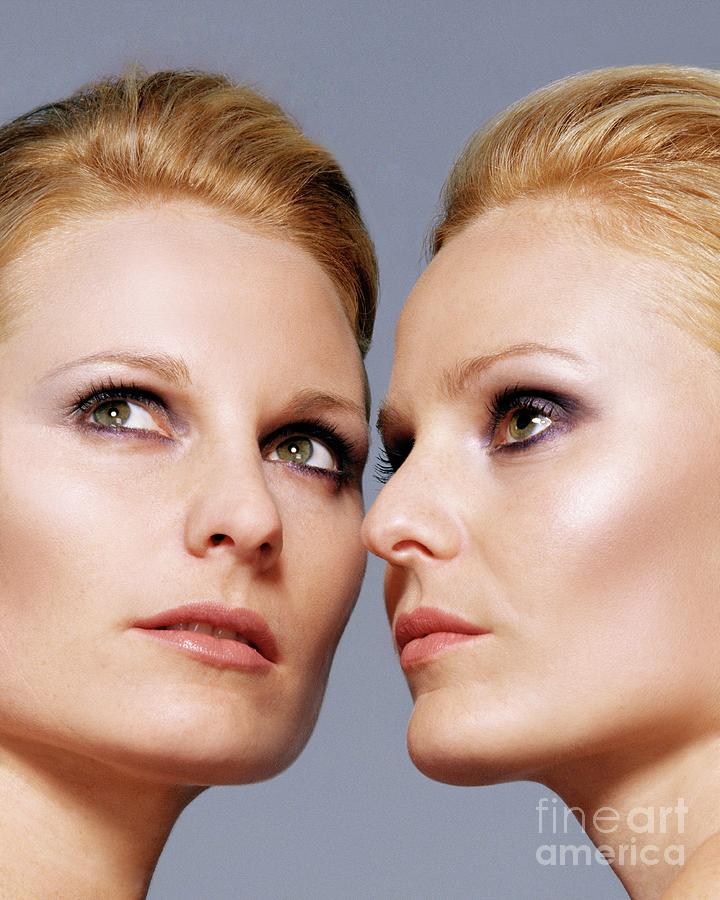This close-up photograph, labeled "Fine Art America" in the bottom right corner, features two women with strikingly similar appearances, both gazing thoughtfully towards the top left corner of the image. The women share distinct features: green eyes accentuated with dark mascara, pink lips, and light blonde to dark blonde hair. Their light-colored eyebrows frame their faces, which exhibit an identical skin tone and detailed makeup. The woman on the left sports light golden or blonde hair and appears deep in thought, her green eyes and makeup conveying a reflective mood. The woman on the right, with slightly lighter strawberry blonde hair, also wears dramatic makeup and has a sharp angular nose and high cheekbones. Both women are positioned very closely to each other against a simple greyish-blue gradient background, emphasizing their entranced expressions as they look towards the same direction, creating a unified sense of contemplation and intrigue.